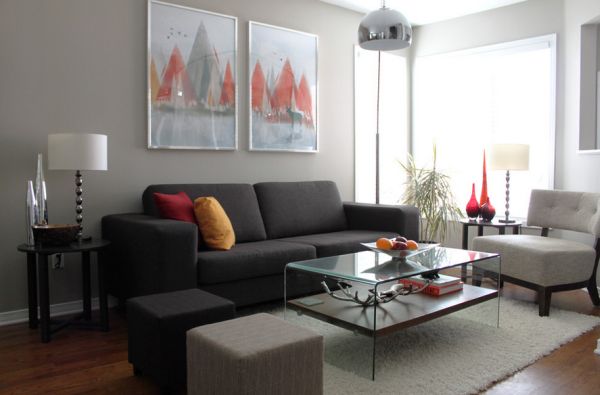This image depicts a meticulously staged modern living room, bathed in natural light from expansive, bright windows on the left side. A gray wall hosts two paintings of abstract, tree-shaped figures in fall hues of red, yellow, and gray. Directly beneath them, a dark gray fabric couch adorned with a vibrant yellow pillow and a red pillow serves as the room's focal point. 

Flanking the couch is a small end table with a sleek drum shade lamp and some glass decorative vases. In front of the couch, a glass coffee table with two shelves rests on a plush white shag rug. The coffee table is adorned with a bowl of fruit and books on its lower shelf. To the left, black and gray cubic ottomans contrast sharply with the lighter elements of the room.

On the right side, a white modern lounge chair with a wooden base and a gap between the seat and the back contributes to the minimalist aesthetic. This carefully curated room, with its clean lines and cohesive design, exemplifies contemporary home decor, possibly suggesting a model home or a setting prepared for guests. A dome-shaped silver chandelier centered over the coffee table completes the elegant and inviting atmosphere.